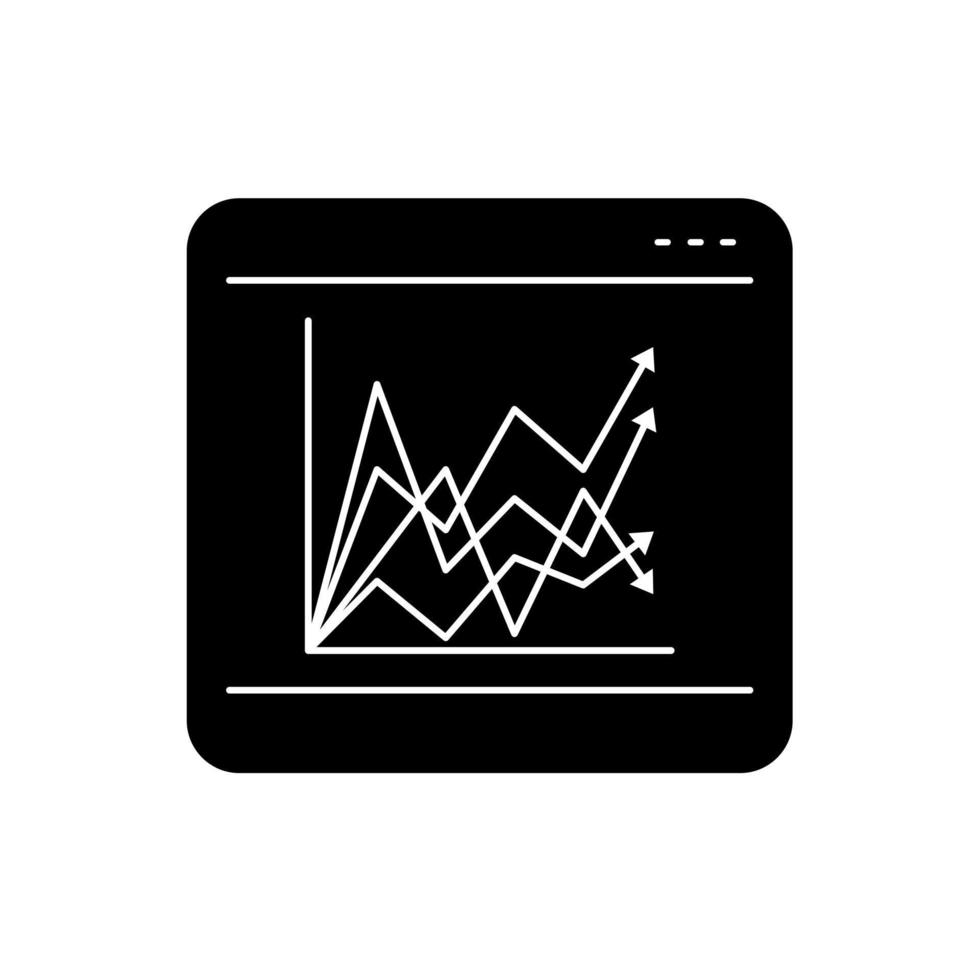This high-quality image features a meticulously detailed black square graphic with white lines and symbols. Dominating the top and bottom edges of the square are two parallel horizontal white lines. Between these lines, the main visual feature is a series of sharp, mountain-like peaks formed by white squiggly lines that ascend and descend in a repetitive pattern. Each peak and trough is accentuated with arrows at their ends, pointing both upwards and downwards, representing fluctuating directions. These squiggly lines, four in total, trace varying paths: the first two rise, the third plunges steeply, while the fourth attempts an awkward ascent but leans towards a decline. Additionally, a prominent white right angle, resembling an 'L' shape, encapsulates these fluctuating lines. In the top right corner of the graphic, there are three small, evenly spaced white dashes. The overall image reflects no text and is presented with exceptional clarity.